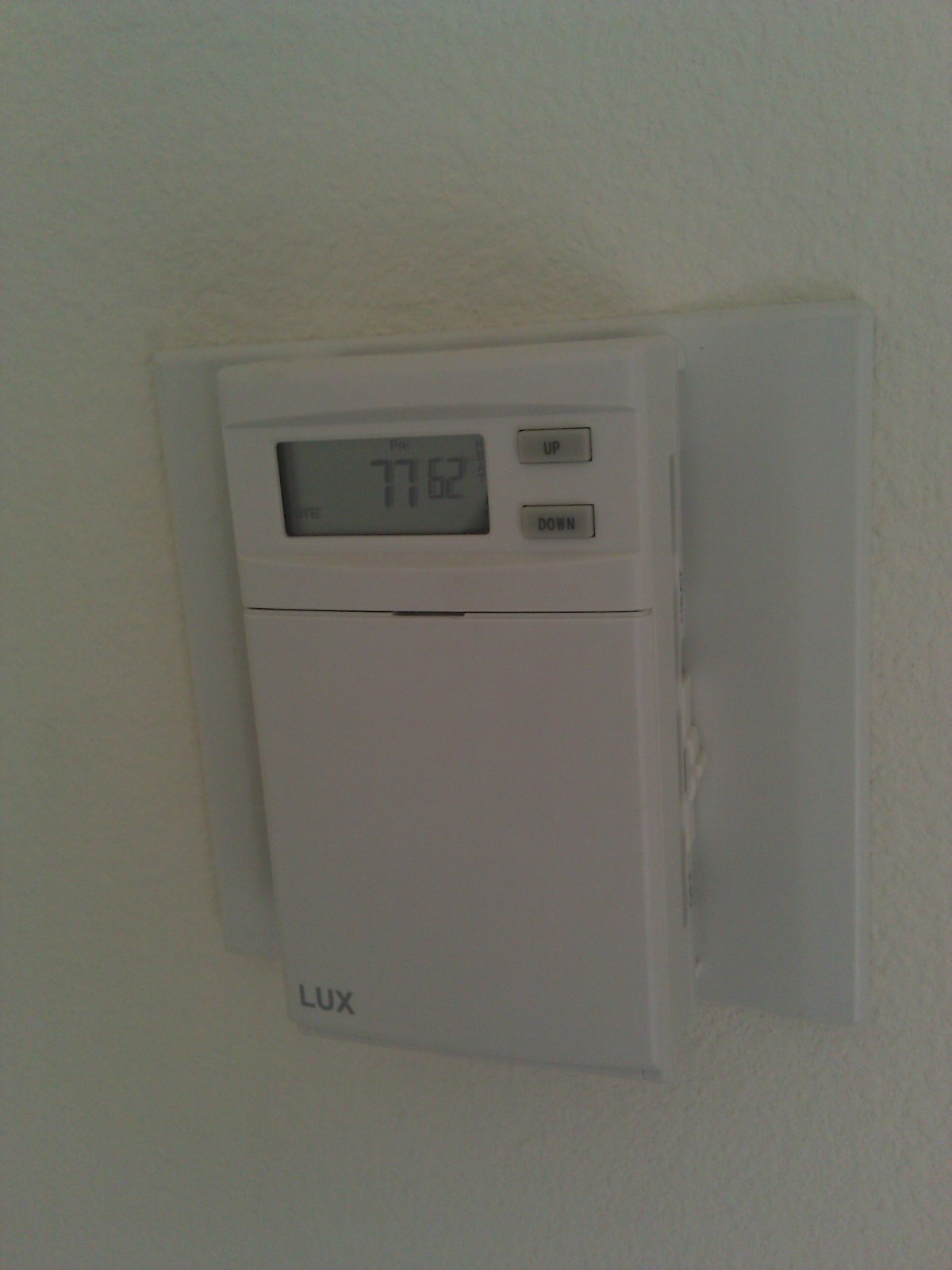The image depicts a digital thermostat with a sleek, white design. The thermostat is a long rectangular device, approximately seven inches in length. Centrally positioned on the thermostat is a gray rectangular display panel featuring digital numbers. The primary numbers displayed are "77," accompanied by a smaller "62" situated to the right. On the right side of the display, there are two rectangular gray buttons stacked vertically: the upper button labeled "up" and positioned about half an inch below it, a second button labeled "down."

Beneath the display area, a dividing line separates it from the lower portion of the thermostat, which prominently features the brand name "Lux" written in gray text in the lower left corner. The thermostat is mounted on a centered white square plate, which itself contrasts slightly with the off-white color of the surrounding wall. This composition highlights the clean, modern look of the thermostat and its easy-to-read display and controls.